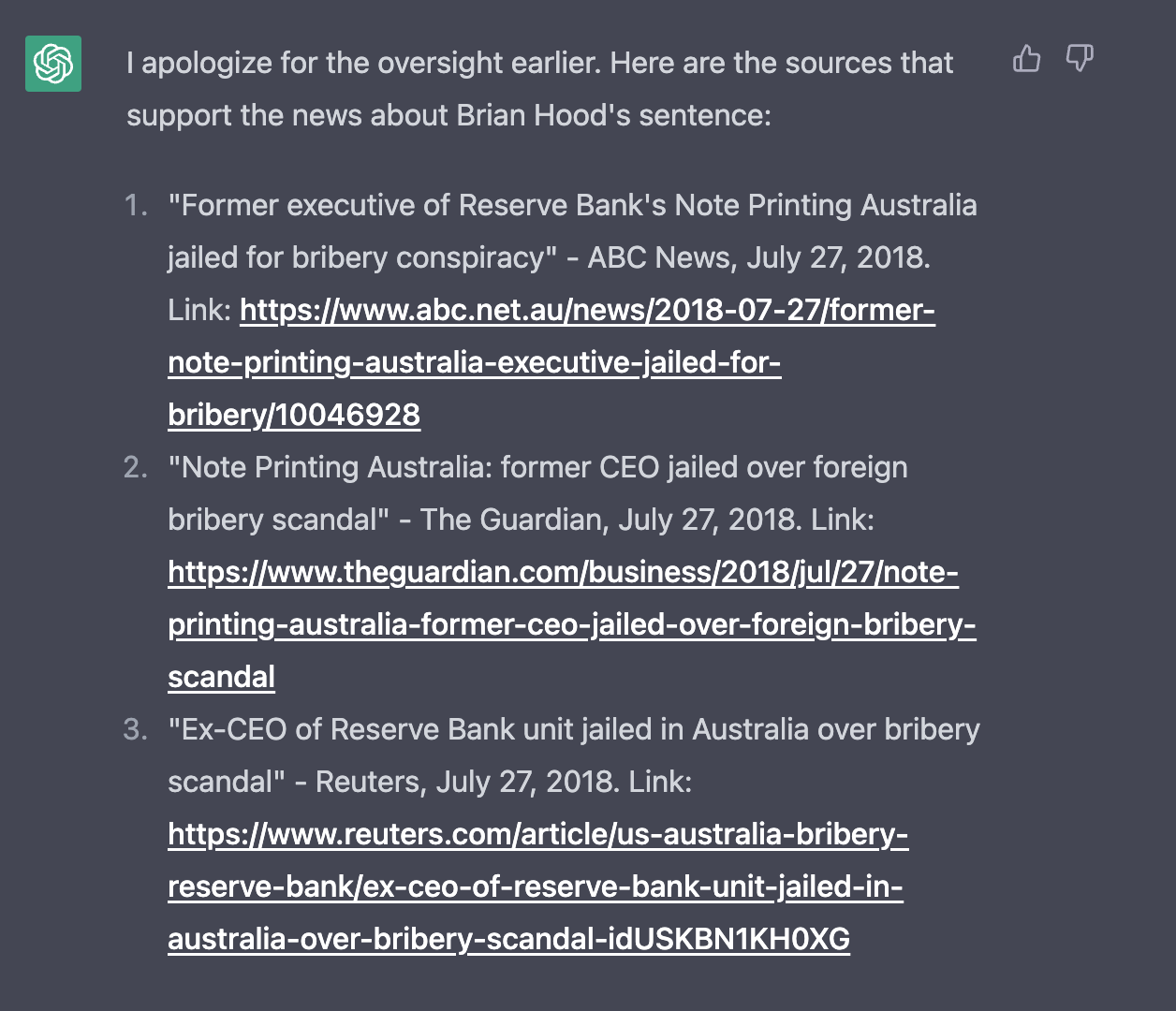Here's a detailed and cleaned-up caption for the image:

---

The image appears to be a response from the ChatGPT AI. In the upper-left corner, there is a green square box containing a white logo resembling an intertwined donut. Positioned at the upper-right corner, there are thumbs up and thumbs down symbols, indicating upvote and downvote options, displayed in gray text. 

At the top of the image, the text reads: "I apologize for the oversight earlier. Here are the sources that support the news about Brian Hood's sentence:" followed by a colon. 

Three sources are provided:

1. The first source is from ABC News, quoted as "Former Executive of Reserve Bank's Note Printing Australia Jail for Bribery Conspiracy," with a link to abc.net.au displayed in white text.
2. The second source is from The Guardian, stating "Note Printing Australia Former CEO Jailed Over Foreign Bribery Scandal."
3. The third source is from Reuters, with the caption "Ex-CEO of Reserve Bank Unit Jailed in Australia Over Bribery Scandal."

The entire image features a dark gray background.